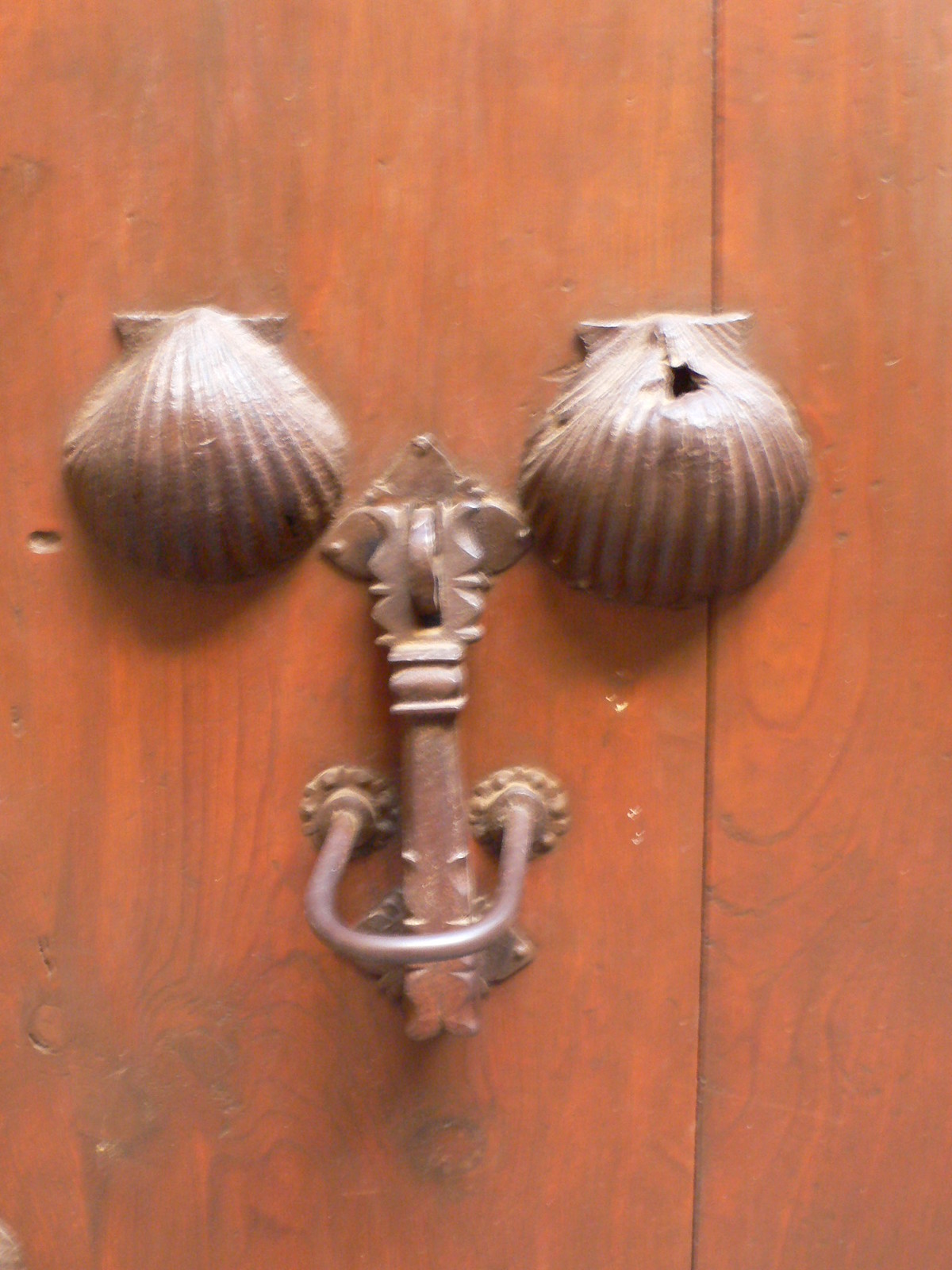In this close-up image, we see an antique wooden door with a dull red tone, devoid of any glossiness. Centrally mounted on the door is an ornate metal door knocker composed of several distinct elements. At the top of the knocker, flanking either side, are two bronze seashell-shaped decorations with intricate veining, resembling clamshells. These seashells appear almost like eyes, adding a decorative touch to the setup. Below them, a straight metal bar with a flower-like design at the top extends vertically, culminating in a horseshoe-shaped piece that serves as the moveable part of the knocker. The hardware appears to be made of bronze or copper, which complements the antique appearance of the overall design.